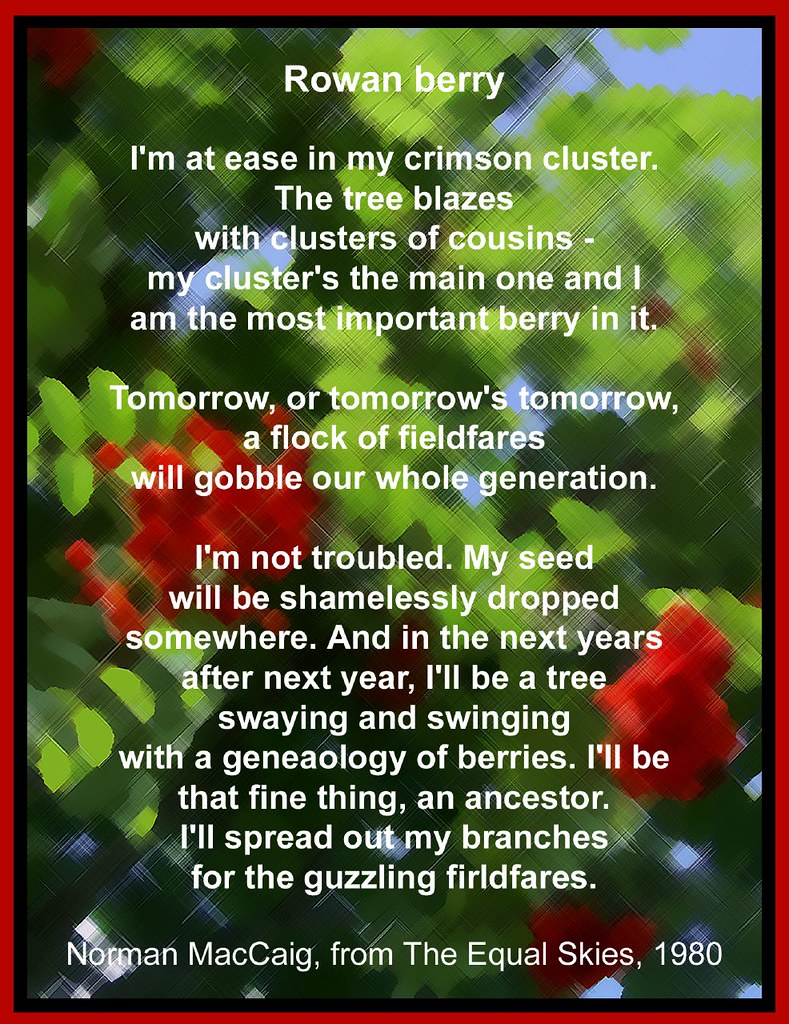The image is a color illustration with a red and black border surrounding it. Inside, the background features an abstract portrayal of red roses and green foliage with a bit of blue sky peeking through. Dominating the image, white text presents a poem titled "Rowan Berry" at the top, followed by the poetic lines: "I'm at ease in my crimson cluster. The tree blazes with clusters of cousins - my cluster's the main one, and I am the most important berry in it. Tomorrow or tomorrow's tomorrow, a flock of field fairs will gobble our whole generation. I am not troubled; my seed will be shamelessly dropped somewhere. And in the next year, after next year, I'll be a tree swaying and swinging with a genealogy of berries. I'll be that fine thing, an ancestor. I'll spread out my branches for guzzling frigid airs." At the bottom of the text, a credit reads "Norman McCaig, from The Equal Skies, 1980." This piece combines typography and illustration to deliver an inspirational message through both visuals and words.